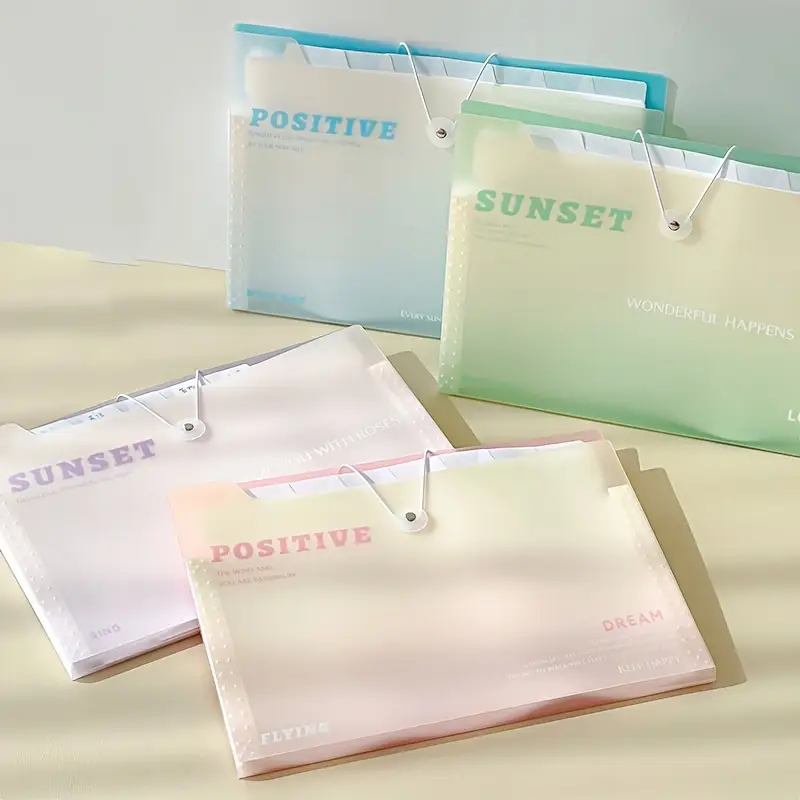In the image, there are four colorful file folders arranged on a light tan table against a white wall. On the left, a light blue (almost turquoise) folder stands upright with the word "positive" written in turquoise letters, secured by a white string closure. In front of it to the right, a light green folder, also upright, bears the word "sunset" and features a similar white closure. Laid flat on the table are two other folders: a pink one on top with the word "positive" in pink letters, overlapping a light purple folder underneath that is labeled "sunset". The overall mood of the image is light and organized, with the colors and texts of the folders creating a cohesive visual arrangement.